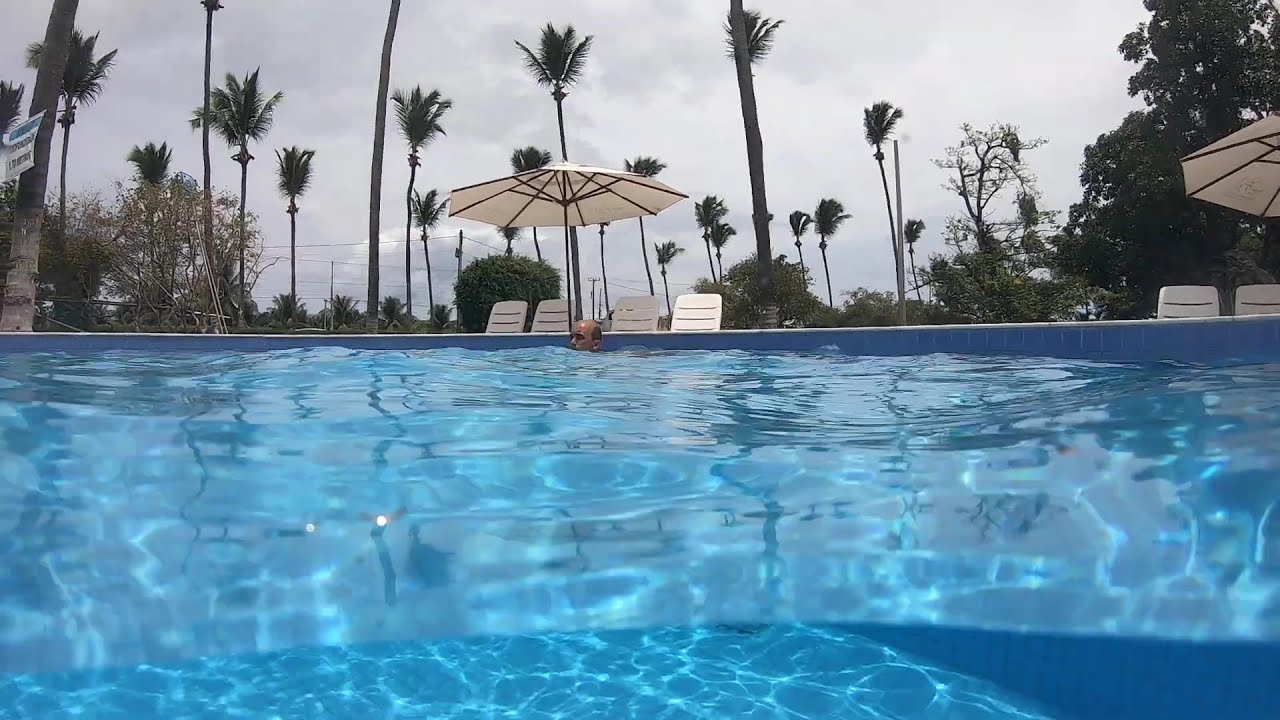From the perspective of the corner of a square-shaped, crystal-clear swimming pool, the photo captures the serene scene almost level with the water. The water displays hues of dark blue and light teal, with gentle ripples surrounding a man with a bald head up to his chin in the water, relaxing against the far corner. Behind him stands a white-topped umbrella centered above four white plastic lounge chairs. To the right, a partial view of another umbrella shades two more plastic chairs. Surrounding the pool area, tall palm trees with high fronds and round, dark green shrubs enhance the tropical atmosphere. Above the scene, the sky is a mix of gray and white clouds, suggesting a rainy day. The setting, likely in a resort-style environment, is tranquil and devoid of other people.